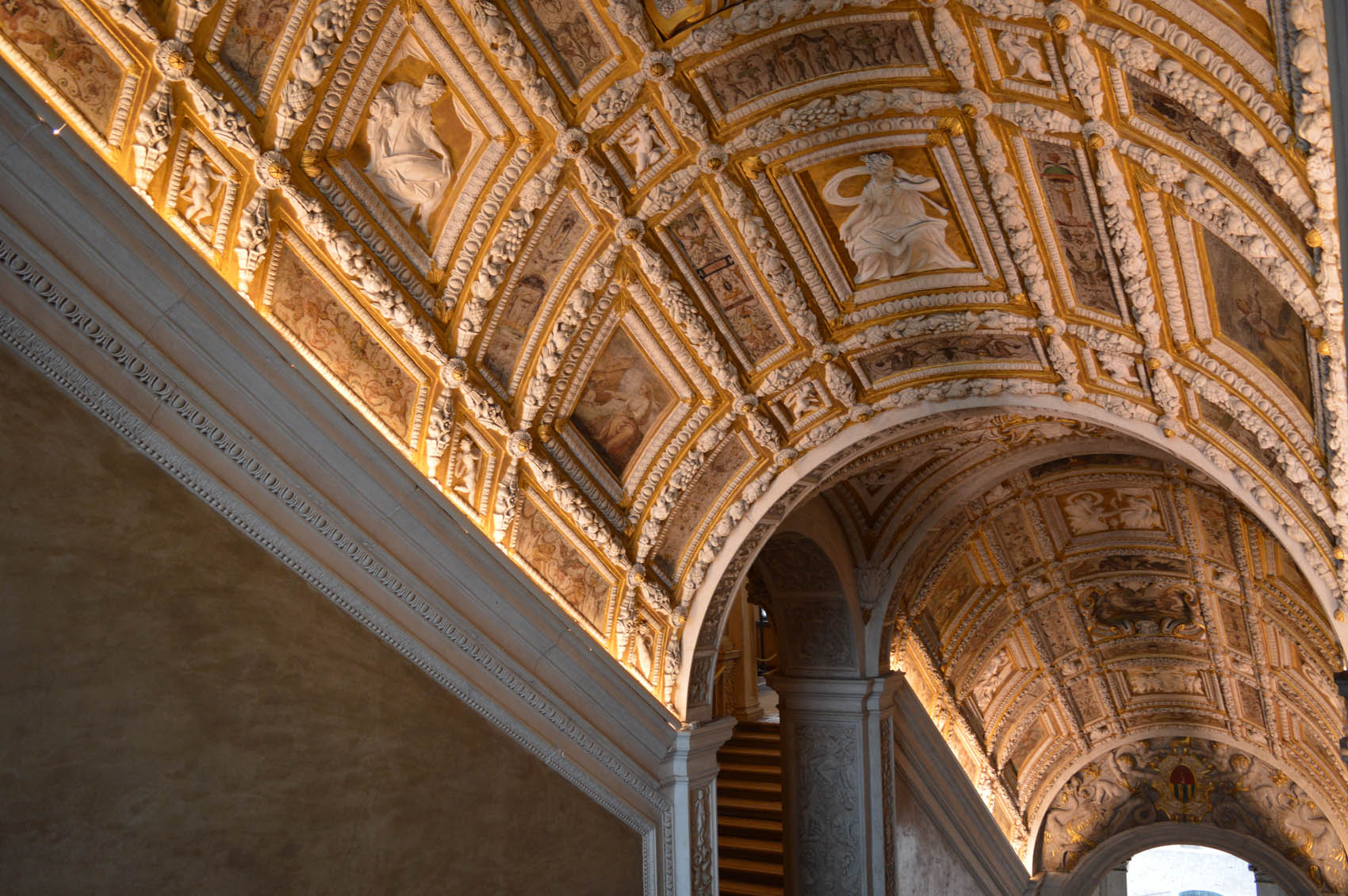The image captures the interior of what appears to be a baroque-style place of worship, possibly a church or temple, characterized by its highly ornate design. The ceiling, which is either dome-shaped or sloped, features a base of gold with intricate white moldings. These moldings are elaborate and detailed, depicting figures of women in robes, framed by borders reminiscent of seashell patterns. The ceiling's rich decoration includes bas-reliefs and engravings that give an impression of marble carved into various patterns and grids, further embellished with artistic illustrations. The photograph is taken from a perspective that emphasizes the grandeur of the ceiling, highlighting the intricate details and marble-like statues. Granite walls and detailed pillars add to the opulent atmosphere, with a staircase visible on the left side, suggesting the image was captured from an ascending viewpoint within the structure.